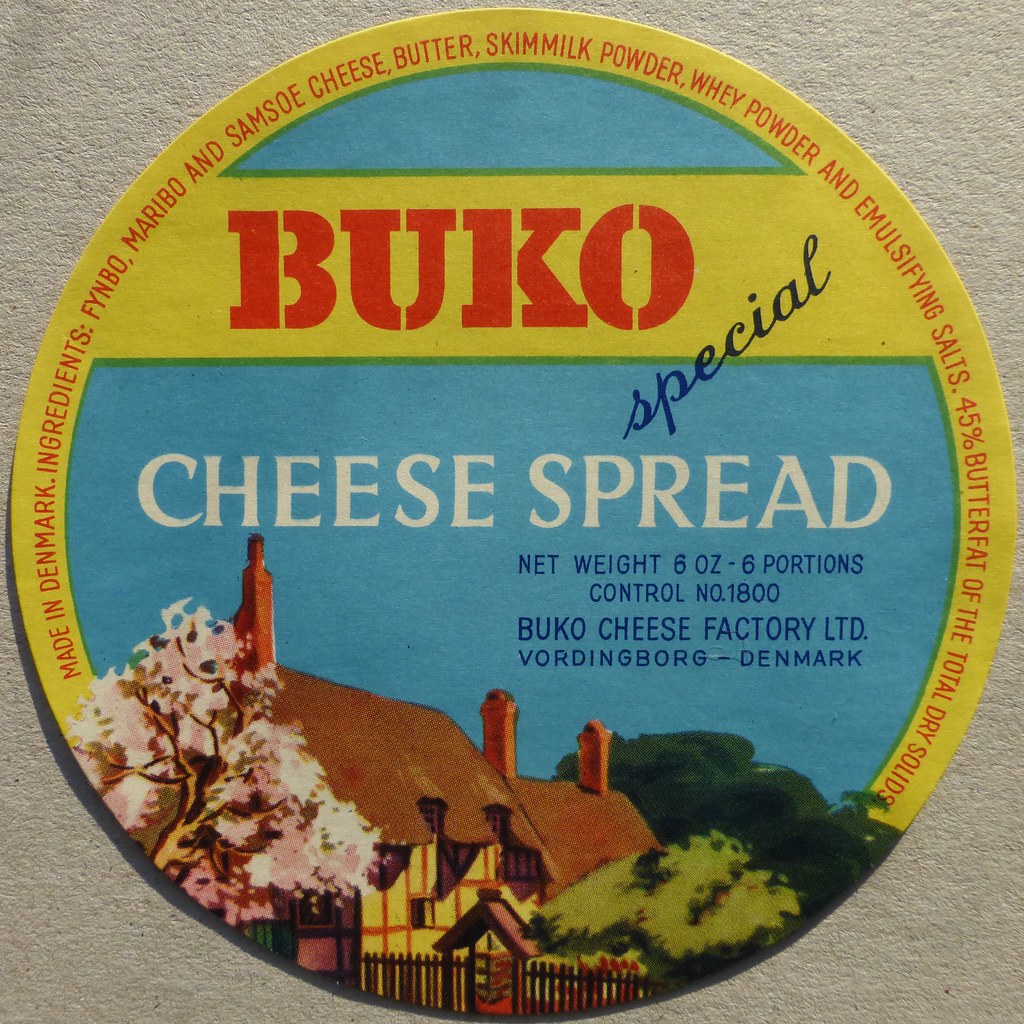This image features a vintage, round paper label for Buko Special Cheese Spread from Vordingborg, Denmark, likely from around the 1970s. The label showcases a yellow border encompassing a bright blue background, indicating a sunny day. Central to the design, the word "Buko" stands out in large, red stenciled letters, with additional details like "Special Cheese Spread" and the net weight (8 oz for 6 portions) prominently displayed across a yellow band in the center.

The bottom section of the label is illustrated with a picturesque scene of Vordingborg, Denmark, featuring an old-style homestead with steep roofs, brick chimneys, and white stucco walls accented by brown wood beams in a checkered pattern. The charming village scene is further complemented by trees, including one adorned with cherry blossoms and another green tree to the right.

Along the edge of the label, detailed information about the cheese spread is provided, listing ingredients such as Fimbo, Marimbo, and Samso cheese, butter, skim milk powder, whey powder, and emulsifying salts, with a butterfat content of 45% of the total dry solids. The label also includes the control number 1800 and identifies the producer as the Buko Cheese Factory LTD in Vordingborg.